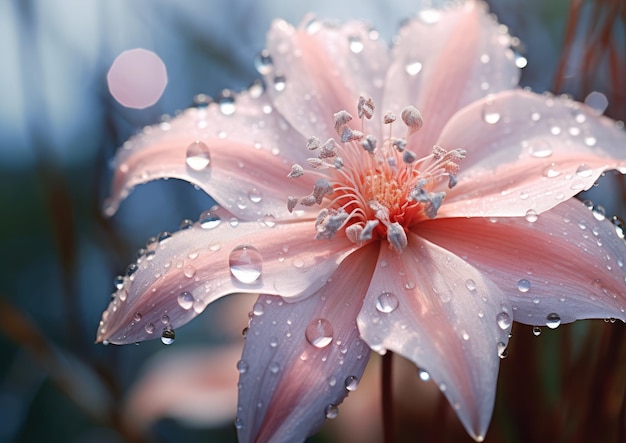The image is a highly detailed close-up of a delicate, soft pink lily, potentially rain-kissed or covered in morning dew. This exquisite flower, which might be real or computer-generated due to its almost too-perfect appearance, features blushing hues towards its center and several tiny, cylindrical droplets of water scattered across its petals. The center of the lily reveals tiny, darker pink stamens. Surrounding the flower, the background is blurred, exhibiting a bokeh effect with a bluish-gray tint, emphasizing the flower as the focal point. Additionally, subtle lens blur and lens flare effects contribute to the composition’s serene and almost ethereal quality.